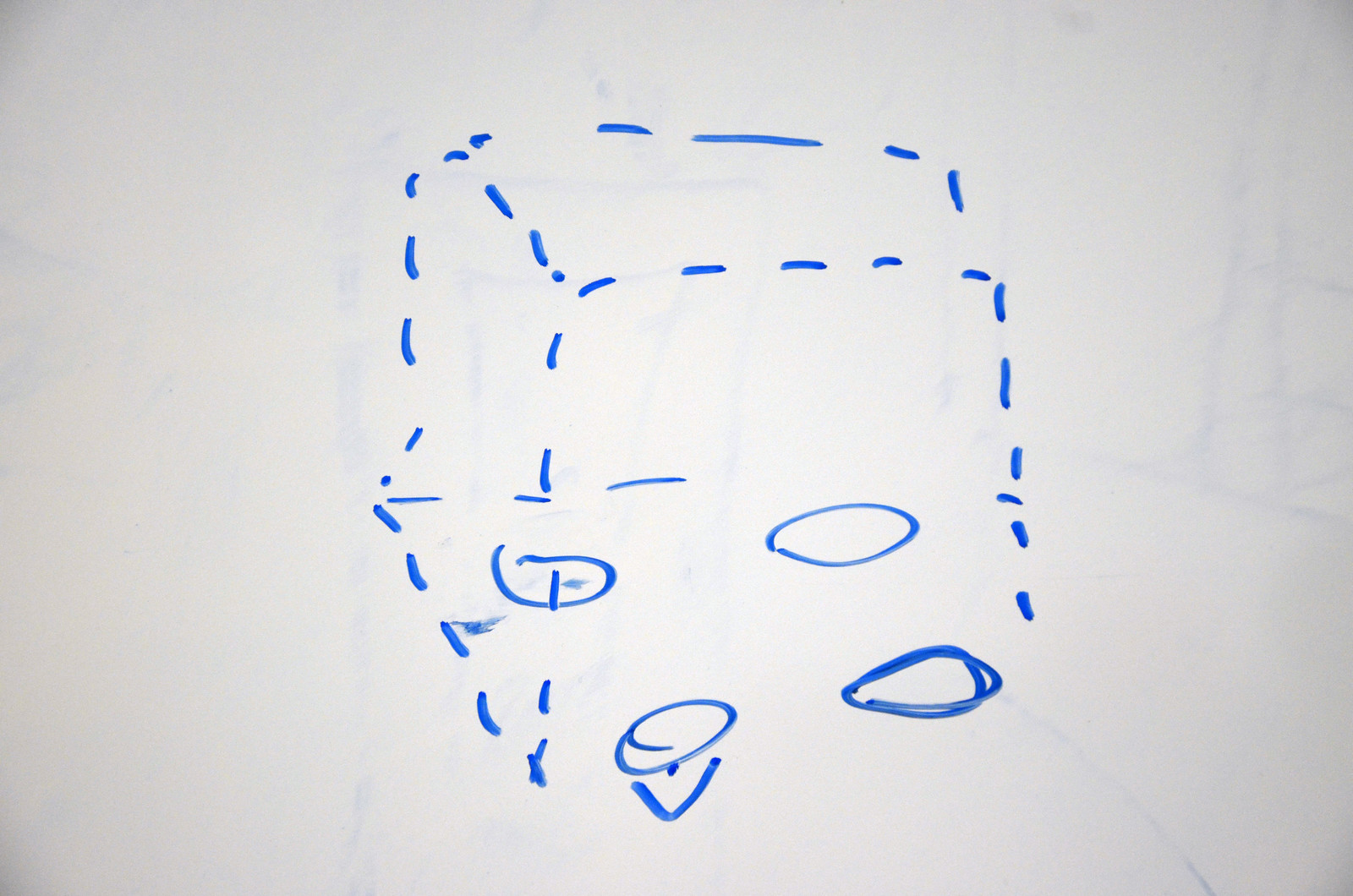This image features a pale blue or grey rectangular background. At the center, there is a roughly sketched cube, rendered with dashed blue lines that give the impression of a three-dimensional shape, though some lines are incomplete or missing. The cube is devoid of any written text on its visible sides and top. The bottom face of the cube displays four hand-drawn circles and a shape resembling the head of an arrow, all rendered in a similarly sketchy style. While the incomplete lines and lack of numbers make it difficult to definitively identify, the four circles suggest that this could be an attempt to depict a die. However, the overall sketchy presentation leaves room for interpretation.